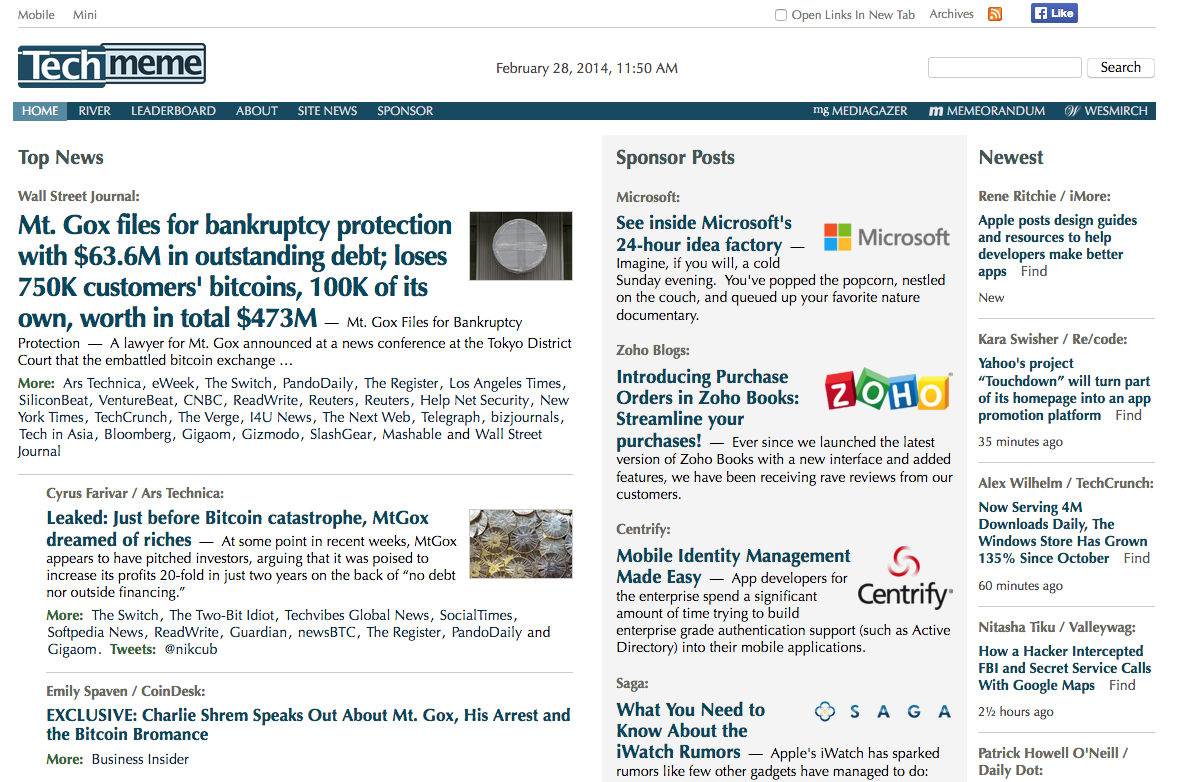A user is exploring a webpage with multiple open tabs, dated February 20, 2014, at 11:50 AM. The search interface shows various categories, including archives, tech articles, and top news. The prominent news story features Mt. Gox, detailing a press conference about financial protection involving significant amounts of money: $63.6 million, $750,000, and $500,000. The total worth is noted as $475,000. The coverage includes links to the Wall Street Journal, media mentions by Miranda Westbridge, and commentary by lawyer Brent Gorski. This descriptive summary captures a snapshot of the user's digital environment, emphasizing the significant information about the Mt. Gox financial news.